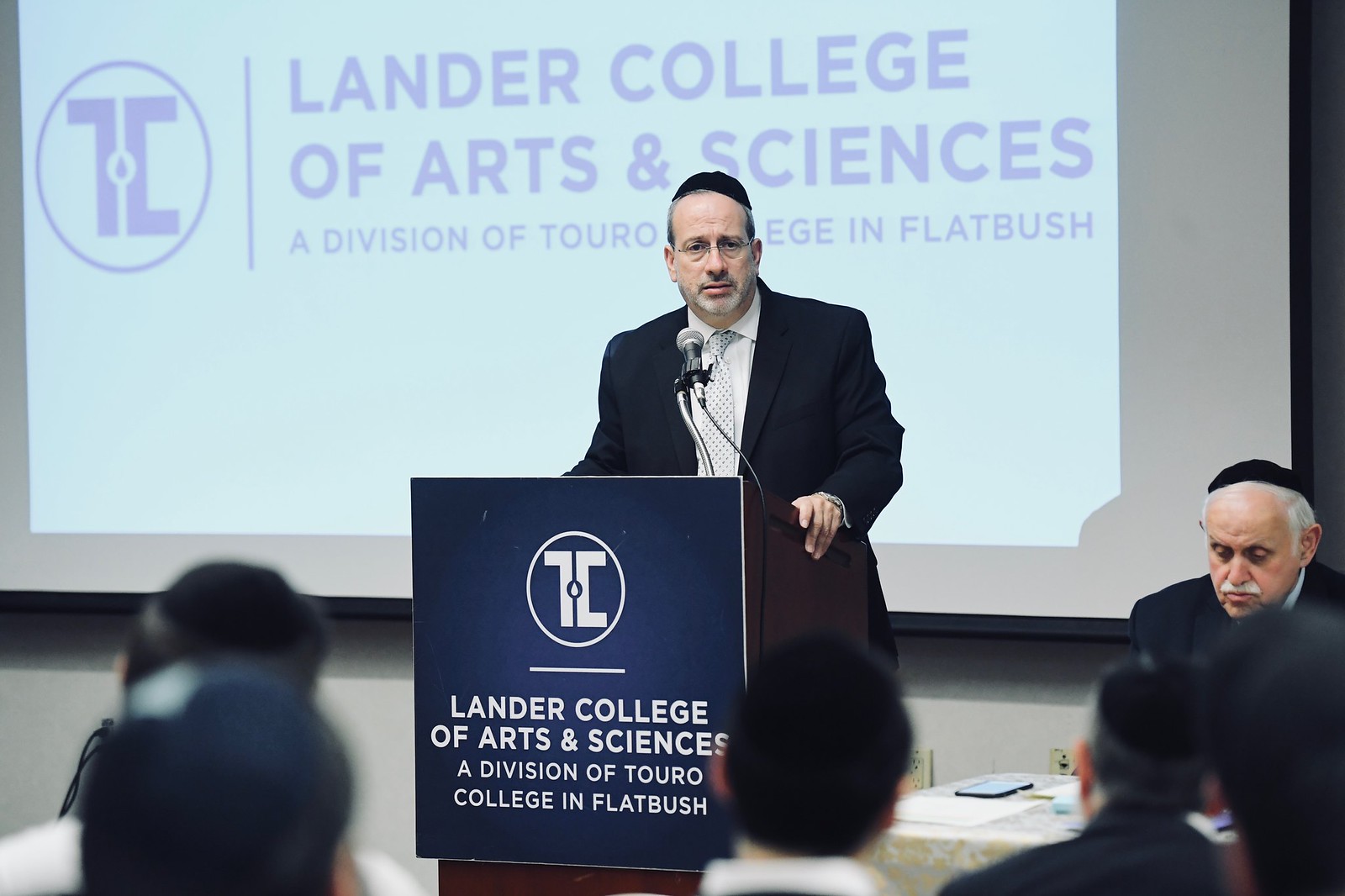In this detailed image, a man wearing a black suit, white button-down shirt, and a polka-dot tie is standing behind a podium, speaking into a microphone. On his head is a religious hat, a yarmulke, indicating he is likely Jewish. The sign on the podium clearly states "Lander College of Arts and Sciences, a division of Touro College in Flatbush," written in white text alongside a symbol resembling an upside-down "L" and a "C" within a white circle. Behind the speaker, a projector screen displays the same text. Another man, also wearing a black suit and yarmulke and distinguished by his white hair and mustache, is seated beside the speaker. The setting appears to be a classroom, where five audience members, also wearing yarmulkes, are attentively watching the speaker, who seems to be engaged with a student, possibly answering a question.